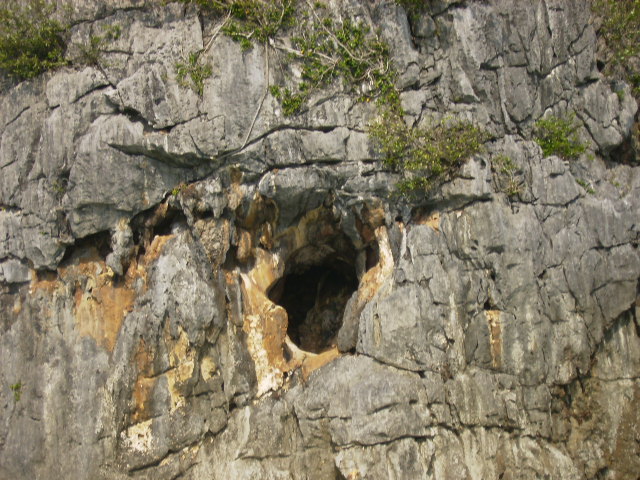The image captures a rugged mountainside dominated by a light gray rock surface interspersed with white streaks and numerous cracks running in various directions. Centered prominently in the image is a small, jaggedly oval cave entrance that stands out due to its distinct coloration—a mix of light brown and white, suggesting either natural staining or mineral deposits. The surrounding rock near the cave transitions into shades of brown and tan, with notable orange and brown scarring towards the bottom left side, possibly due to water and mold. The upper portion of the image features sparse vegetation with branches hanging down, contributing some green to the otherwise barren stone face. Despite the apparent zoom in the photograph, the cave appears difficult to access, perched on a nearly vertical cliff face that offers little in the way of natural handholds or footholds.